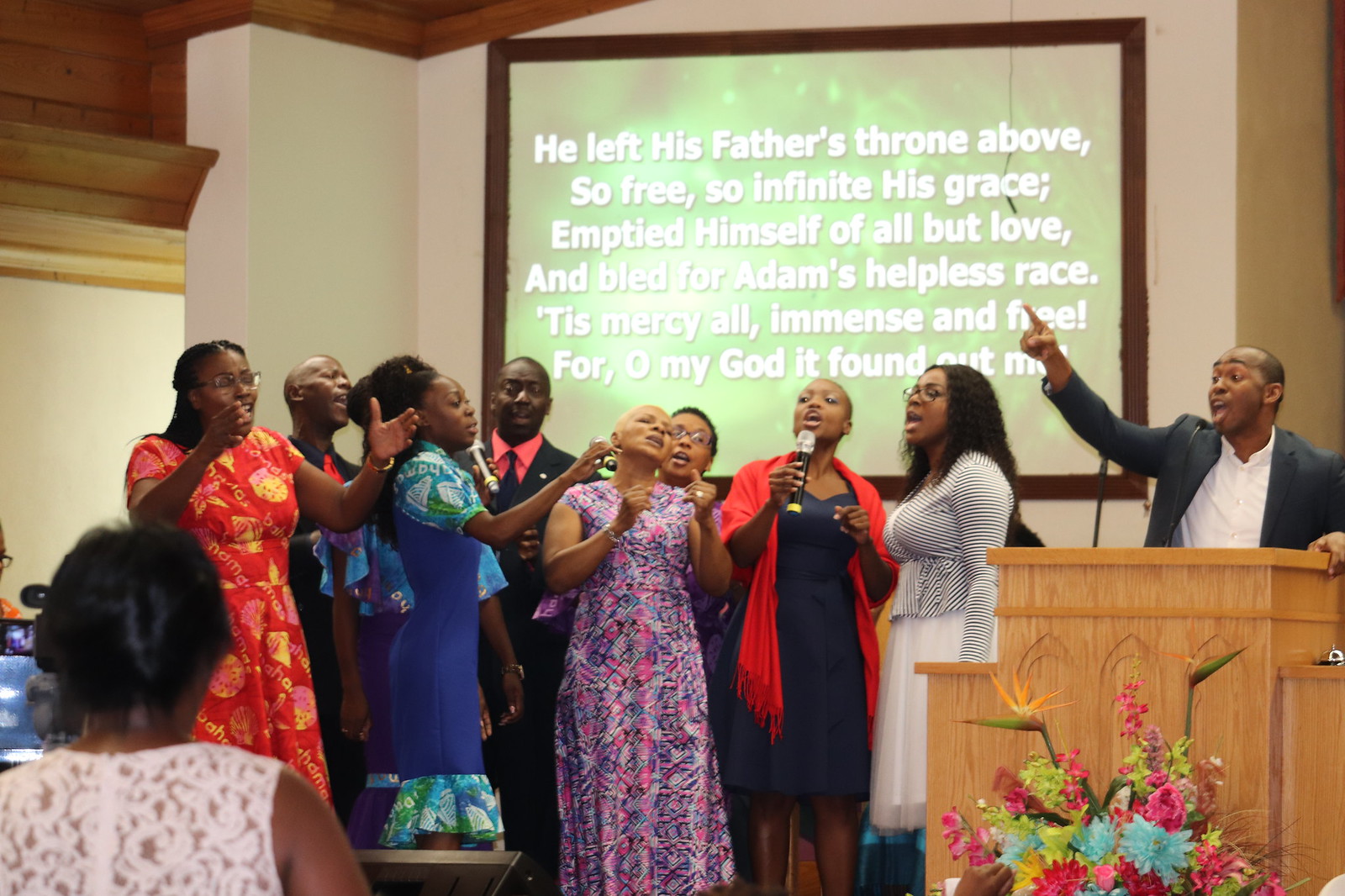This detailed photograph captures a lively moment during a church service. Taken from the perspective of someone sitting in the pews, the image is rectangular and showcases a mid-sermon scene framed in a church setting. On the right side, a middle-aged African-American preacher stands behind the pulpit, passionately pointing upwards with his finger while speaking into a microphone. He is dressed in a black suit jacket and a white shirt, exuding an animated energy. In front of the pulpit is a large bouquet of colorful flowers.

To the left, a group of nine men and women, dressed in their finest Sunday attire, stand on stage. Their hands are raised, and their mouths wide open as they enthusiastically sing, likely a gospel hymn. The congregation in the front row, partially visible from behind, is also standing, fully engaged in the worship.

A projector screen in the background displays the lyrics to a hymn: "He left his Father's throne above, so free, so infinite his grace. Emptied himself of all but love and bled for Adam's helpless race. 'Tis mercy all, immense and free, for oh my God, it found out me." This adds to the communal atmosphere as everyone can follow along.

In the foreground, a woman with her hair pulled up in a bun, dressed in a white lace dress, sits attentively, watching the sermon. The overall ambiance is one of joy and spirited worship, capturing the essence of a vibrant church service.